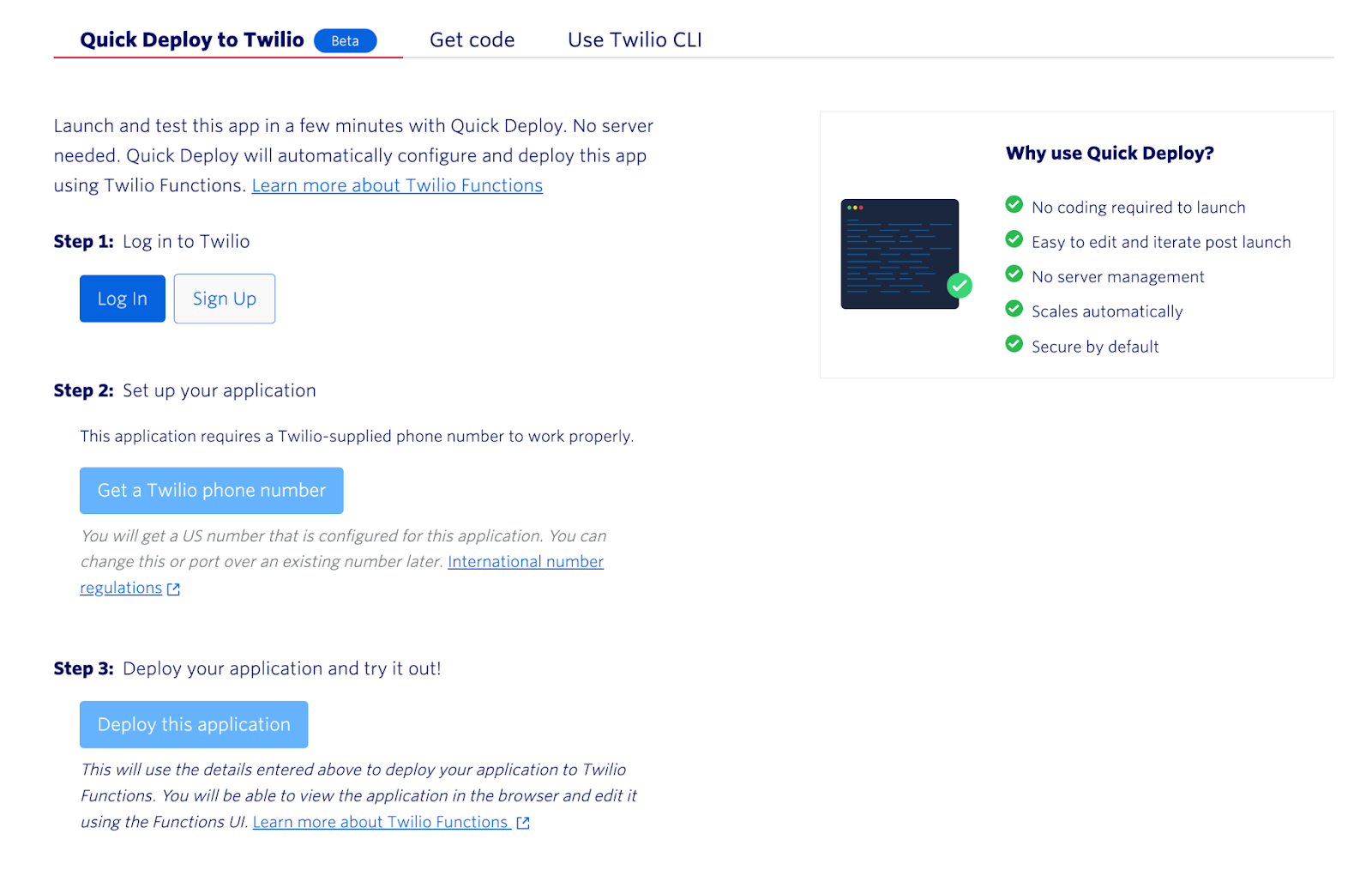This is a detailed screenshot from a PC displaying the Twilio application interface. The focal point of the image is an extra instructions page titled "Quick Deploy to Twilio," prominently featured in bold blue text located in the upper left-hand corner. Adjacent to the title is a blue button with white "Beta" text, indicating that the functionality is in its testing phase. 

At the top of the screen, there are three main options available to the user: "Get Code," "Use Twilio CLI," and "Quick Deploy to Twilio." Below the main title is a step-by-step guide that outlines the process for quickly deploying to Twilio. This instructional content is organized into an introduction followed by a "Step One, Step Two, and Step Three" format.

In the upper right-hand corner, there is a "Why Use Quick Deploy" widget. This section includes a small diagram represented by a black thumbnail with blue lines that symbolize text. Below the diagram, a list of benefits is presented, each accompanied by a green circle with a white checkmark. The listed benefits under the "Why Use Quick Deploy" section are as follows:
1. No coding required to launch
2. Easy to edit and iterate post-launch
3. No server management
4. Scales automatically
5. Secure by default